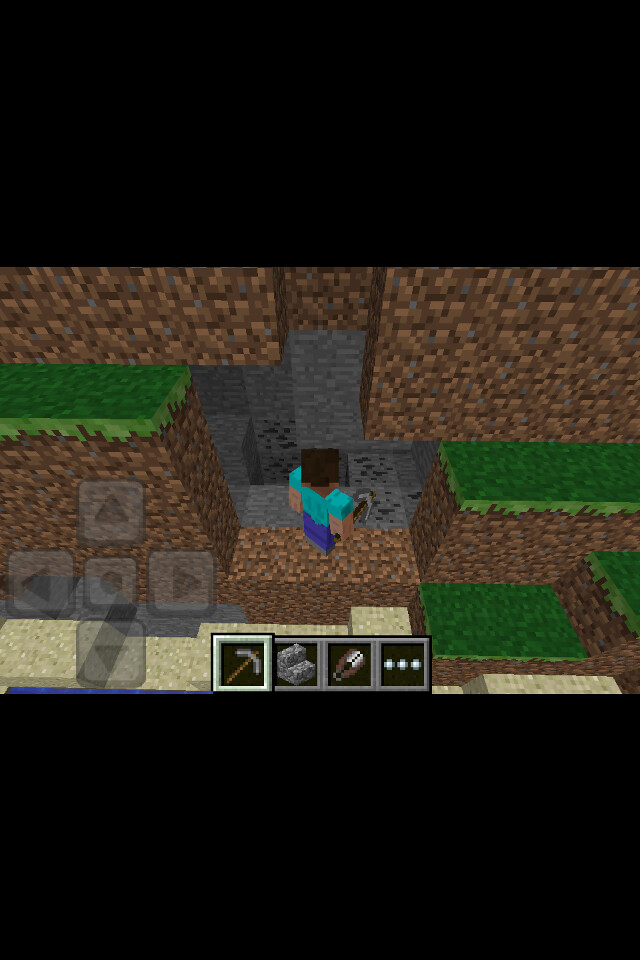The image is a screenshot from a mobile version of Minecraft, likely an iPhone, displayed with black letterbox bars occupying the top and bottom 30% of the screen. In the center of the image, there's a visible overlay of directional pads in the lower left corner, indicating on-screen controls. The character, known as Steve, is positioned centrally, wearing a teal shirt and blue pants, facing roughly one o'clock. He stands on a dirt cliffside flanked by grassy inclines on both sides, with a sandy area below. Steve is depicted in the act of mining into a stone wall, creating a hollowed-out space in front of him. The interface shows four selectable equipment options at the bottom of the screen, including a pickaxe, stone, clippers, and a menu button, signifying it is indeed Minecraft gameplay.